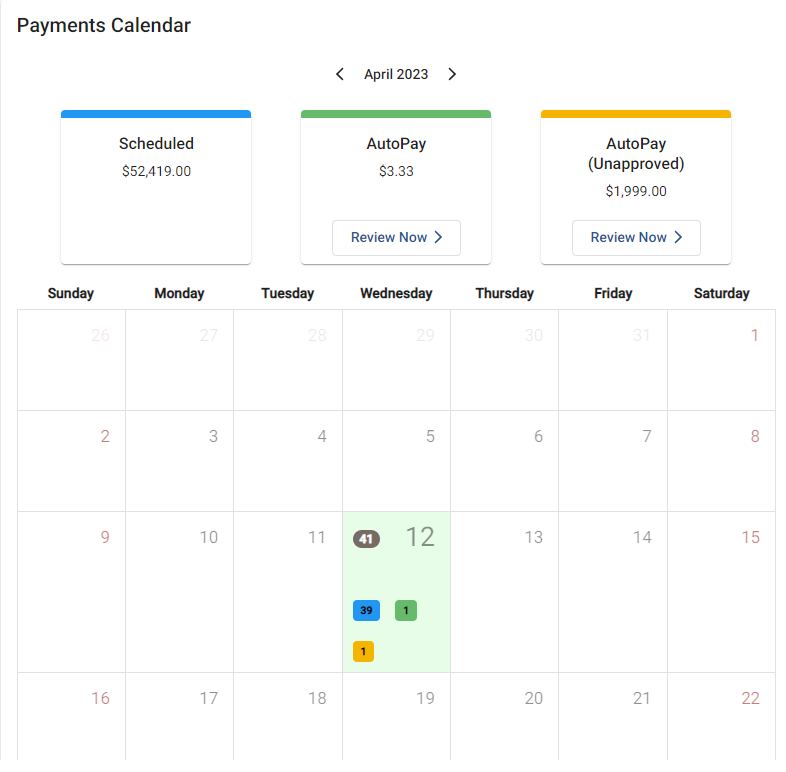This image is a detailed screenshot of a digital payments calendar interface for April 2023, likely displayed on a computer screen. 

In the top-left corner, the title "Payments Calendar" is prominently displayed. At the center of the header, "April 2023" is shown, flanked by navigational back and forward arrows, allowing the user to browse different months.

Beneath the header are three distinct boxes, each providing specific information about various types of payments:
1. The first box on the left is labeled "Scheduled" with a prominent blue line on top. It indicates a total of $52,419 in scheduled payments.
2. The middle box is labeled "AutoPay" with a green line on top, showing a smaller total of $3.33 for automated payments. Below it is a "Review Now" button.
3. The third box on the right, labeled "AutoPay Unapproved," features a yellow line on top and indicates an amount of $1,999 awaiting approval. This box also includes a "Review Now" button.

Below these informational boxes is a calendar grid formatted with seven columns representing each day of the week (Sunday through Saturday) and four visible rows accommodating up to 31 days, depending on the month.

Specifically highlighted on the calendar is the date April 12th, which contains the summary of the payments within color-coded small icons:
- A blue icon labeled "39" representing the 39 scheduled payments.
- A green icon labeled "1" corresponding to the single automated payment.
- A yellow icon labeled "1" representing the unapproved auto payment.

This detailed layout conveys essential financial scheduling information in a clear, organized manner for user review and action.